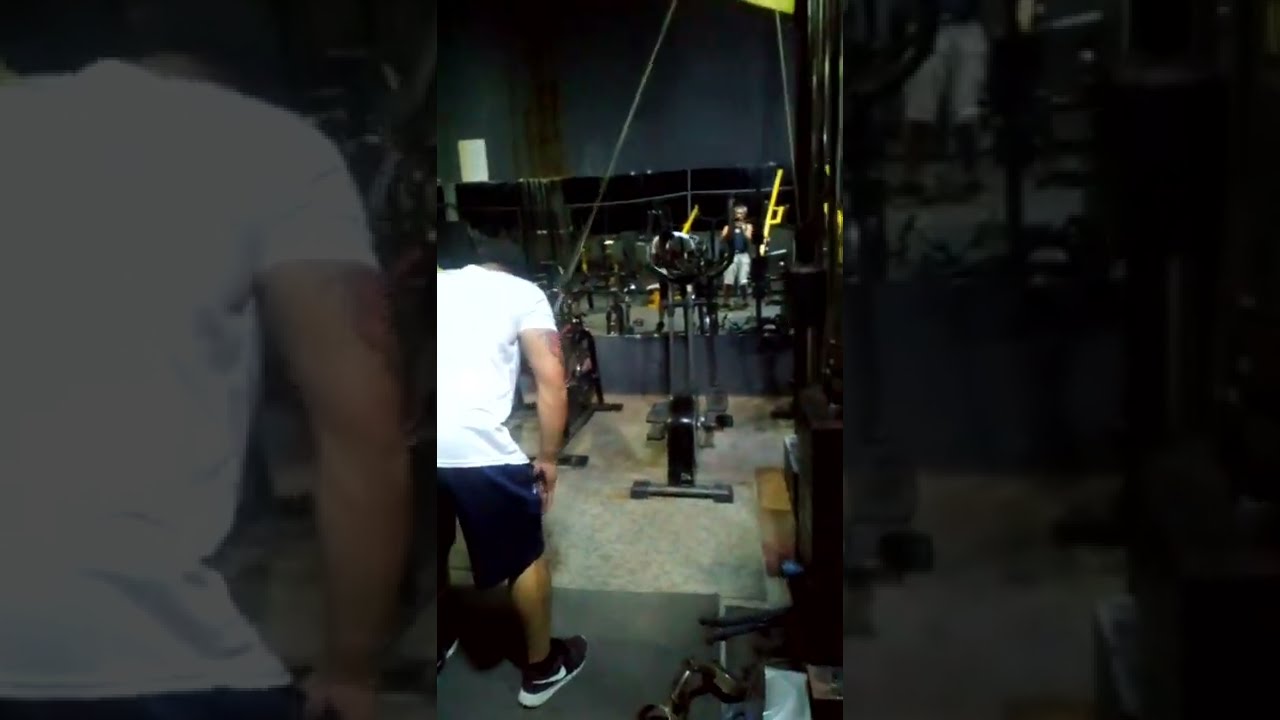In a dimly lit, crowded gym, a man in the foreground leans over, gripping a bar intensely. He wears a white T-shirt, blue shorts, and black Nike sneakers, emblazoned with the iconic white checkmark. His arm features a tattoo. The gym is cluttered with yellow workout machines and features a dark floor and walls smeared with brown smudges. In the background, a child in a black tank top and white shorts raises his hands in front of his face. The scene appears within a video frame, showcasing the same image as an enlarged, darkened backdrop, adding an intriguing layered effect.